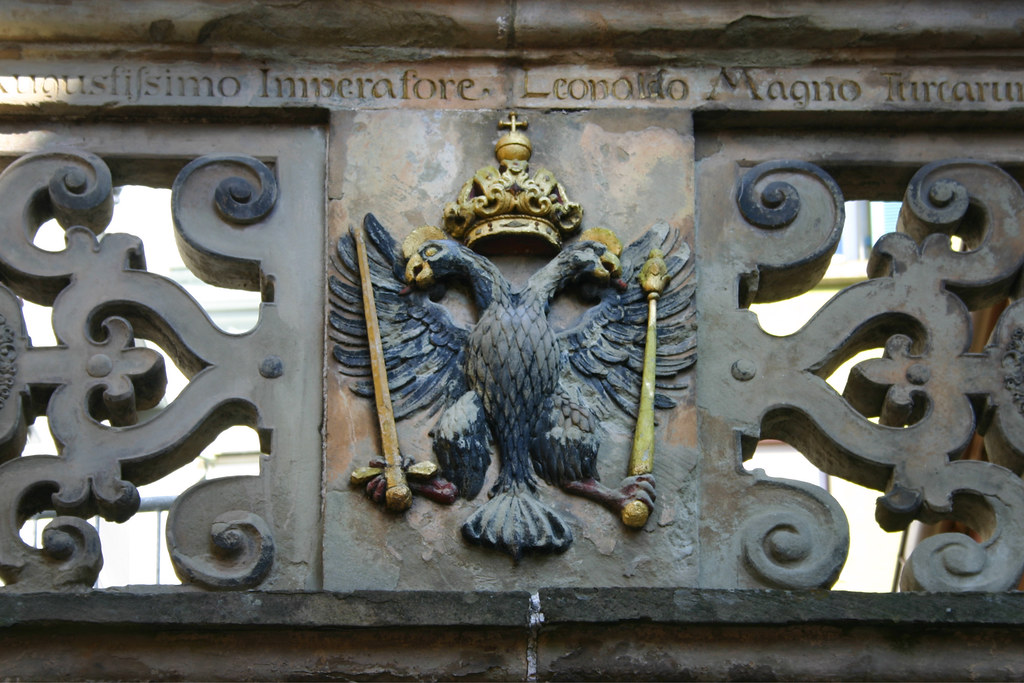In the center of this color photograph, set against the gray stone of an old monument, is a striking, two-headed blue eagle with yellow beaks and crests. Each head looks in a different direction, and the eagle’s outstretched wings and fierce gaze give it a commanding presence. In each claw, the eagle holds an object: the left claw appears to grasp a paintbrush or a saber, while the right claw seems to hold a scepter or drumstick. Above the eagle is a gold-colored crown with a cross on top of it. Further up, inscribed in what might be Italian or Latin, are the words "Imperator," "Leopoldo," and "Mono," though the remaining text is indiscernible. Surrounding the eagle, on either side, are intricate open scrollwork designs, hinting at the architectural details of the building behind it. There are no people or animals present in the photo, highlighting the majestic and solitary nature of the emblem.